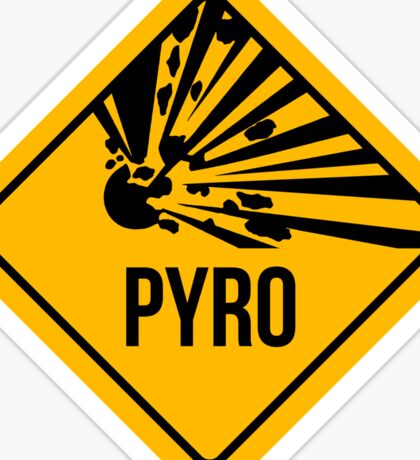The image displays a yellow caution street sign, resembling a diamond shape. The sign is slightly cropped, cutting off the top, bottom, left, and right edges, leaving only the central portion visible. The sign has a layered design: an outer white border surrounding a yellow square, inside which there is a black diamond-shaped outline. Within this black border, the central illustration depicts a black and white explosion, resembling a broken stone or a planet shattering, with fragmented pieces and rays extending outward. Below this explosive design is the text "P-Y-R-O," written in bold, black, uppercase letters.